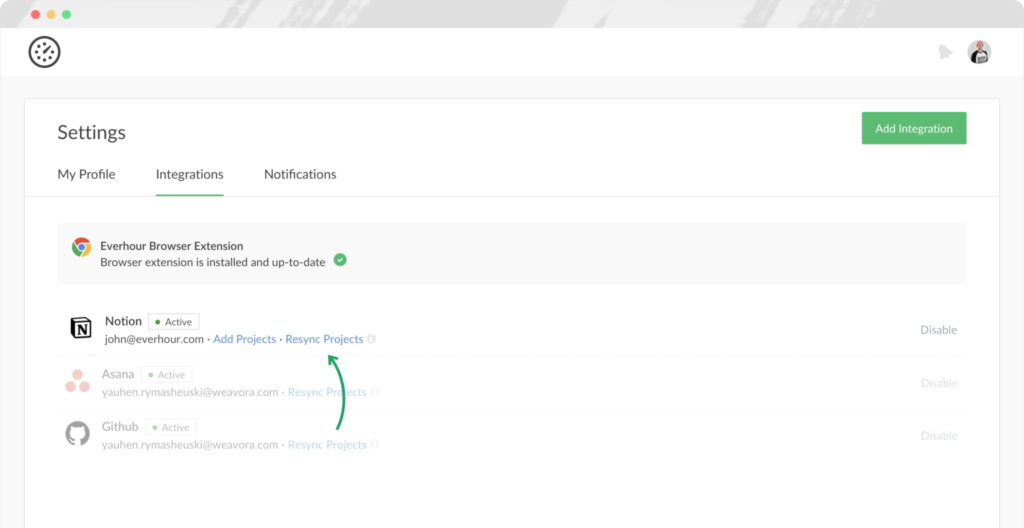The image showcases a detailed settings page interface. At the top, three colored dots—red, yellow, and green—are visible, reminiscent of traffic lights. Below these dots is a circular black logo adorned with a variety of dots, resembling a clock. The page prominently displays "Settings" and features a green "Add Integration" button.

Underneath, the page is divided into several sections with options like "My Profile," "Integrations," and "Notifications." Notably, the "Integrations" section is highlighted by a green line, indicating it is selected. This section lists multiple integration options, beginning with the "EverHour Browser Extension," which is marked with a Chrome logo. To the right of this entry, a green check mark confirms that the browser extension is installed and up to date.

Following the browser extension are three additional integrations:
1. **Notion**: Displays the associated email, john@everhour.com, alongside two buttons— "Add Projects" and "Re-sync Projects." A green arrow points towards the "Re-sync Projects" button.
2. **Asana**: Indicates the status as "Active" and includes a "Re-sync Projects" button.
3. **GitHub**: Also marked as "Active," featuring a "Re-sync Projects" button.

The overall design features a white background, with colorful buttons and additional options providing a visually appealing, user-friendly interface.